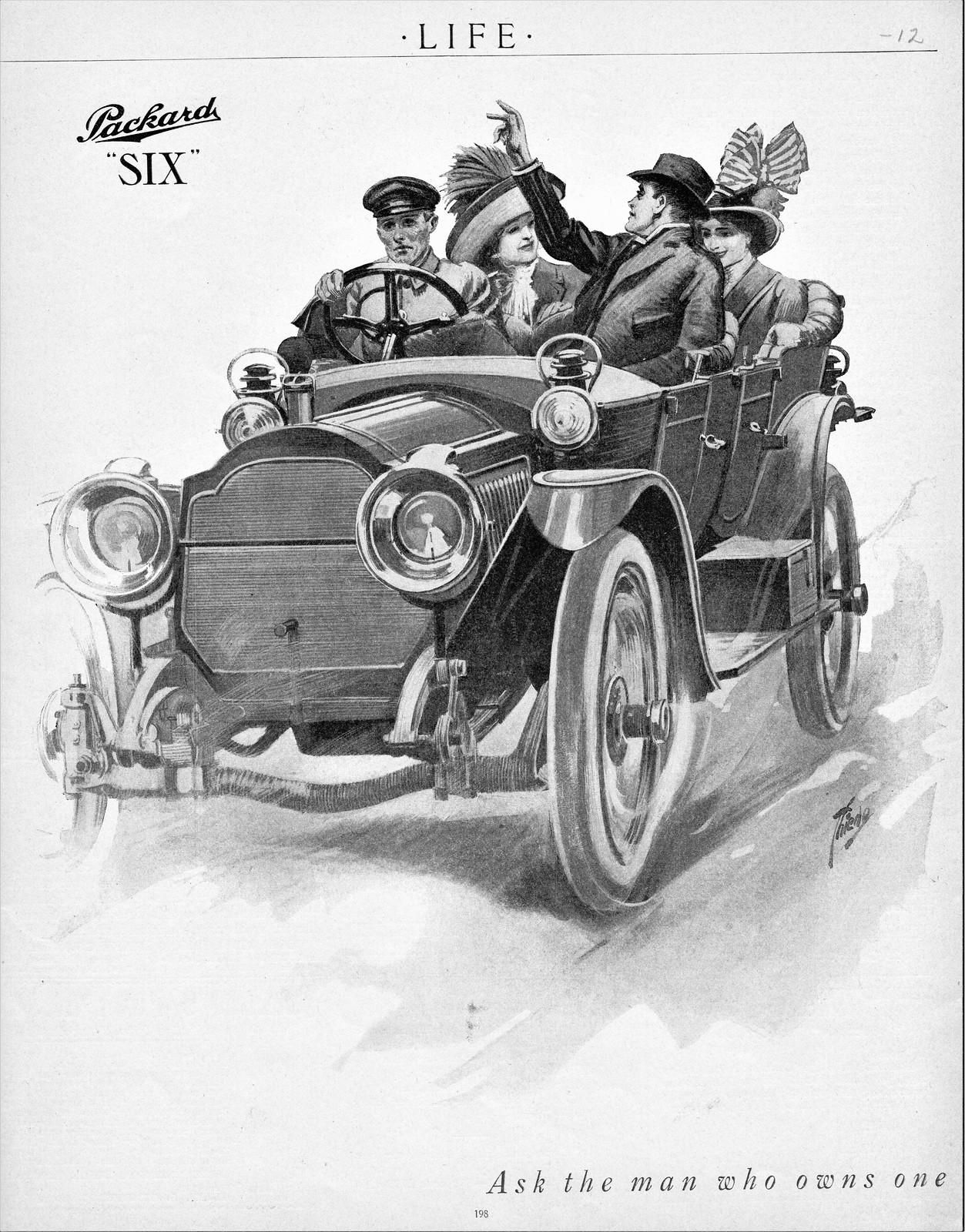This detailed black and white advertisement features a highly realistic grayscale sketch of a vintage Packard 6 car. The car, depicted with the top down and thin wheels indicative of its era, is chauffeured by an impeccably dressed driver. The chauffeur, clad in a uniform reminiscent of the early 20th century, drives as a suited man with a hat rides alongside him in the front passenger seat, gesturing with his arm raised. In the spacious back seat, two elegantly dressed women with large, ornate hats sit comfortably. The image suggests a scene from the early 1900s, possibly the 1930s. The advertisement includes prominent text: "Packard 6" in the upper left-hand corner, "Life" at the upper center, and the slogan "Ask the Man Who Owns One" in the lower right-hand corner. Additionally, the upper right-hand corner bears a handwritten note in pencil reading "minus 12." This artwork, likely from Life Magazine, underscores the luxury and sophistication associated with owning a Packard 6.